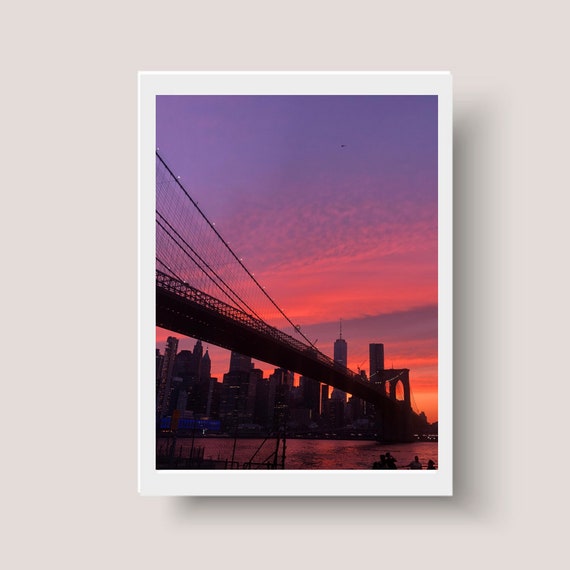This image features the iconic Brooklyn Bridge captured during a captivating evening sunset. Presented within a white, Polaroid-like frame against a strikingly light lilac square background, the photograph draws immediate attention to the bridge's dark, silhouetted structure. The sky is an enchanting blend of pink, orange, and purple hues, streaked with delicate white clouds as the sun sets, casting a serene glow over the scene. The bridge extends from the upper left center to the right corner, with visible suspension lines adding to its majestic presence. Below, the river reflects hints of pink from the colorful sky above. In the lower right corner, a small group of onlookers is visible, taking in the breathtaking view, while the backdrop is adorned with towering skyscrapers and luminous buildings, adding depth and life to the evening cityscape.